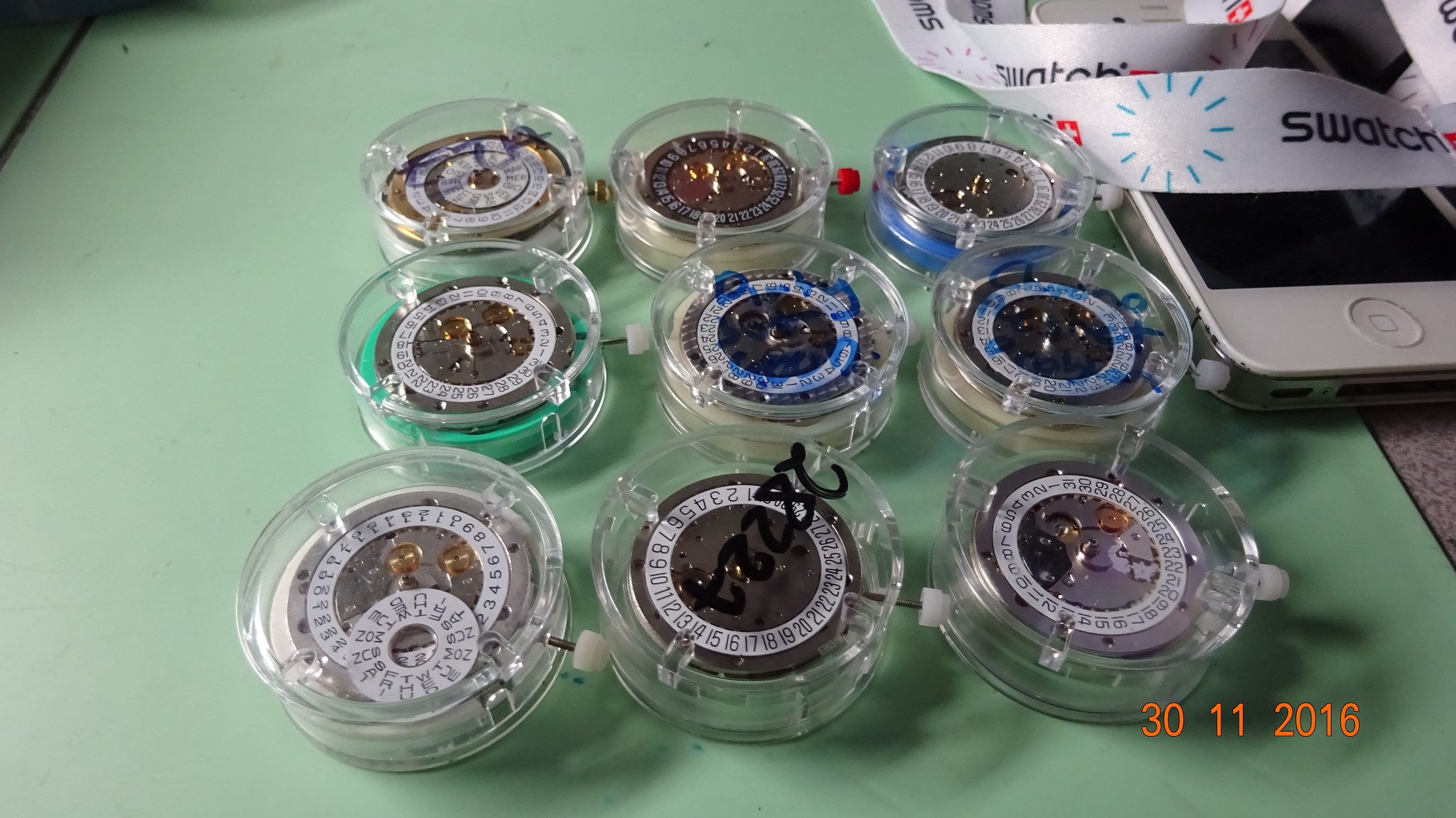The image showcases multiple watch components and clear cases, arranged in a 3x3 grid, all part of the Swatch collection. They are resting on a green Borco mat, with an iPhone and a Swatch-branded ribbon, resembling a lanyard, positioned in the top right-hand corner. The clear cases contain various watch parts in gold and silver, with visible numbers that seem to go up to 30. Light enters from the left, casting shadows to the right, and some watch dials extend slightly from the cases. A date, "30-11-2016," is noted in the bottom right-hand corner of the image.